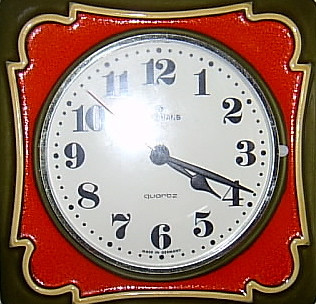This square photograph, framed in a sleek black border, showcases a classic round analog wall clock. The clock itself features a pristine white face adorned with elegant black numbers in a sophisticated font, and minute markers encircle the periphery, allowing for precise time-telling. Currently indicating 4:19, the clock is encased in a shiny black rim and protected by a glass dome, enhancing its vintage appeal. The photo, taken with a flash, reveals a pronounced light flare at the center, obscuring the clock's brand name. Surrounding the clock is an eye-catching, glossy red frame with intricately designed corners, adding a touch of decorative flair to the composition.